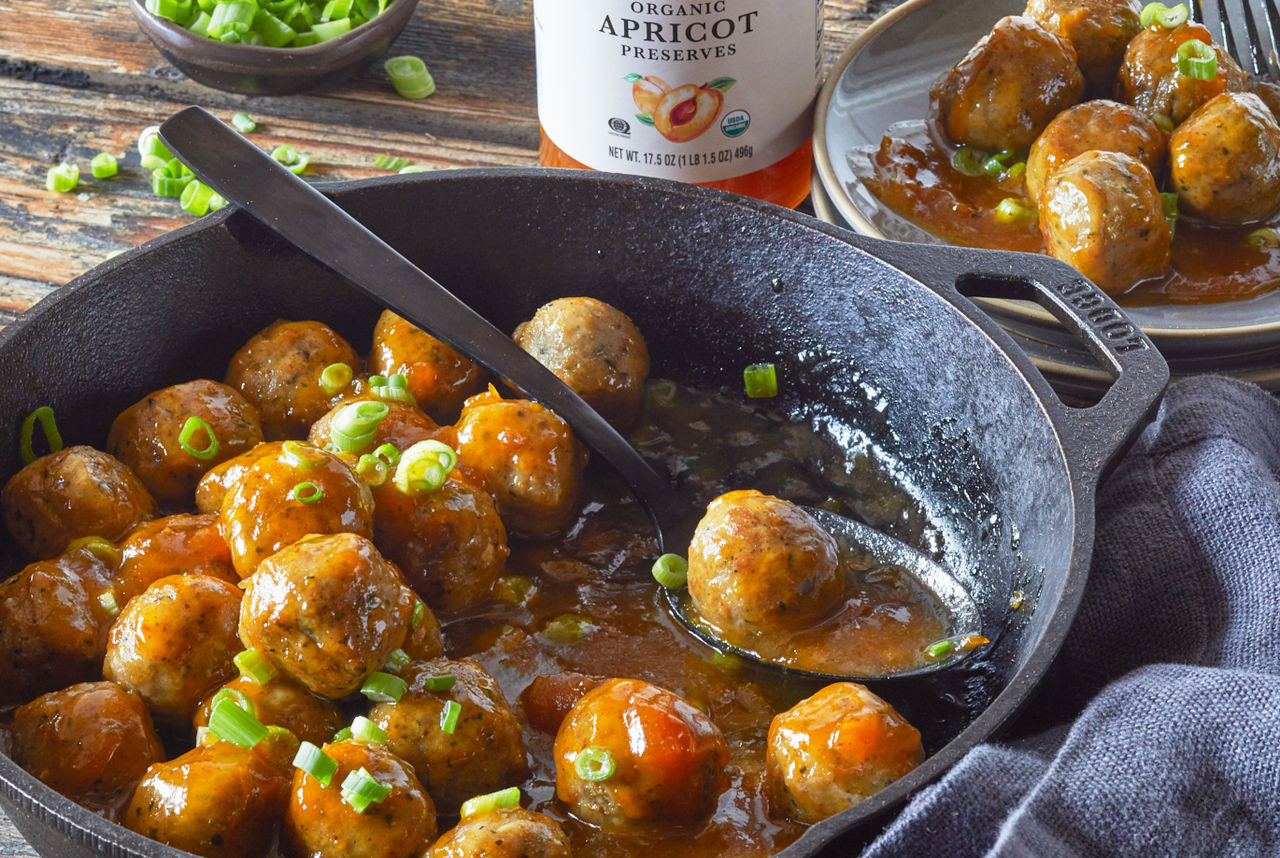In this professionally arranged, detailed close-up food photograph, a centerpiece meatball rests in a black cast iron Lodge skillet, bathed in an enticing orange sauce and garnished with finely chopped green onions. Dominating the image, the skillet hosts numerous similarly garnished meatballs, creating a mouth-watering scene. A spoon in the center cradles a single meatball drenched in the same sauce, emphasizing the dish's texture and presentation.

In the top left corner, part of a small bowl brimming with additional chopped green onions is visible, adding a fresh green accent to the composition. Slightly higher in the frame, the bottom of a jar labeled "organic apricot preserves" hints at the sweet and savory base of the sauce. The jar, adorned with images of apricots, stands out with its orangey liquid contents.

On the top right, a gray plate set atop additional plates holds a pile of meatballs, echoing the skillet’s generous portion. The tip of a fork peeks from the very corner, suggesting readiness to savor the dish. The skillet is set atop a blue cloth, folded and placed on a rustic, dark brown wooden table, completing the homely and inviting setting of this culinary creation.